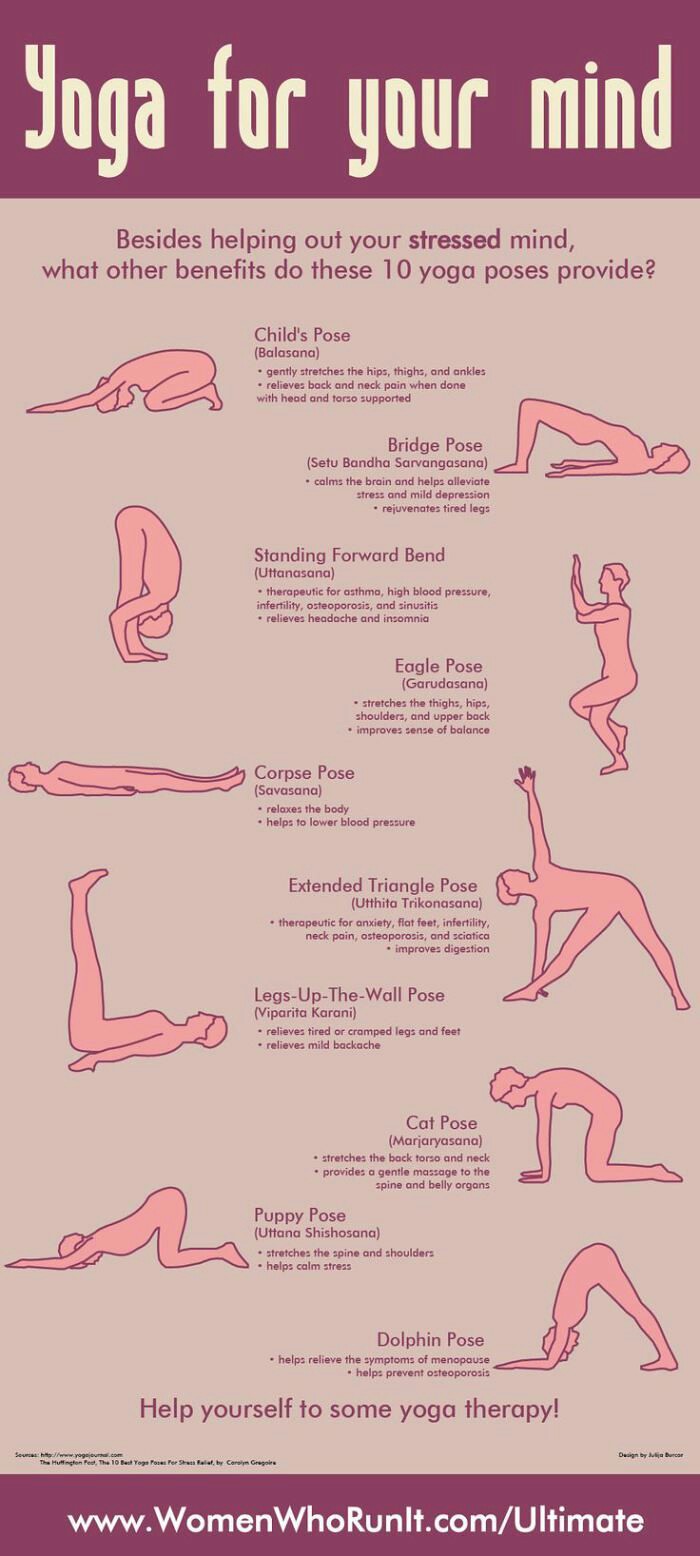The poster is a detailed graphic illustration showcasing "Yoga for Your Mind". At the top, a maroon bar with cream-colored letters titles the poster. Below the title, it reads: "Besides helping out your stressed mind, what other benefits do these 10 yoga poses provide?" 

Down the right and left edges of the page, there are images of ten different yoga poses, five on each side. These images are pink silhouettes of a person demonstrating each pose. In the center of the page, there is a column of text detailing each pose's name and benefits.

The poses featured include:
- **Child's Pose**: Gently stretches the hips, thighs, and ankles. Releases back and neck pain when done with support.
- **Supported Bridge Pose**: Soothes the brain, alleviates stress and mild depression, and refreshes tired legs.
- **Standing Forward Bend**: Therapeutic for asthma, high blood pressure, infertility, osteoporosis, arthritis, headache, and insomnia.
- **Eagle Pose**: Stretches the thighs, hips, shoulders, and upper back. Enhances balance.
- **Corpse Pose**: Relaxes the body, and helps lower blood pressure.
- **Extended Triangle Pose**: Therapeutic for anxiety, flat feet, infertility, neck pain, osteoporosis, sciatica, and improves digestion.
- **Legs Up the Wall Pose**: Relieves tired and cramped legs, and mild headache.
- **Cat Pose**: Stretches the back, torso, and neck, providing a gentle massage to the spine and abdominal organs.
- **Puppy Pose**: Stretches the spine and shoulders, calming stress.
- **Dolphin Pose**: Helps relieve symptoms of menopause, prevents osteoporosis, and provides therapeutic benefits.

At the bottom, another maroon banner with white letters reads: "www.womenwhorunit.com ultimate."